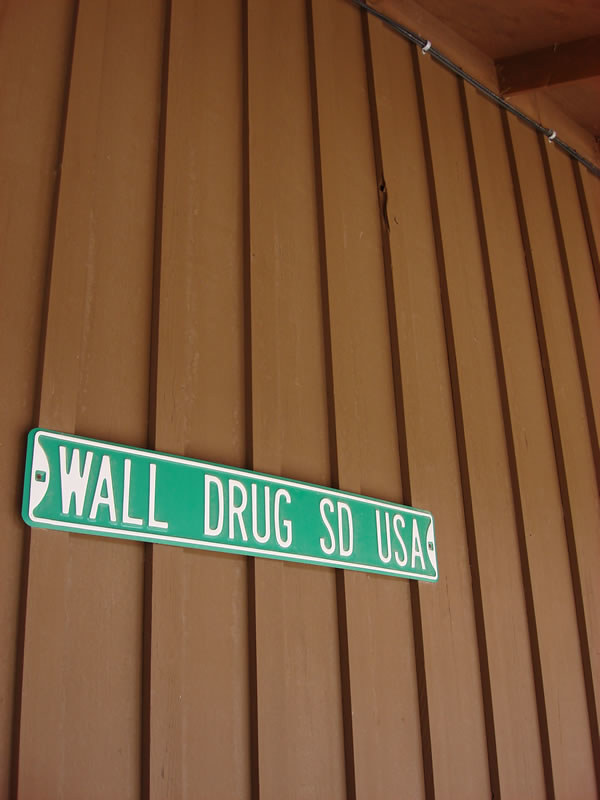This image features a green street sign that reads "Wall Drug SD USA," securely nailed to a brown paneled wooden wall. The wall consists of horizontal wooden slats, artfully stacked one over the other, contributing to a rustic aesthetic. Above the sign, a long black string or wire runs beneath a deck, adding a subtle detail to the composition. The ceiling boasts a prominently visible darker brown beam, which might be made of wood or steel, further enhancing the structural charm of the scene.